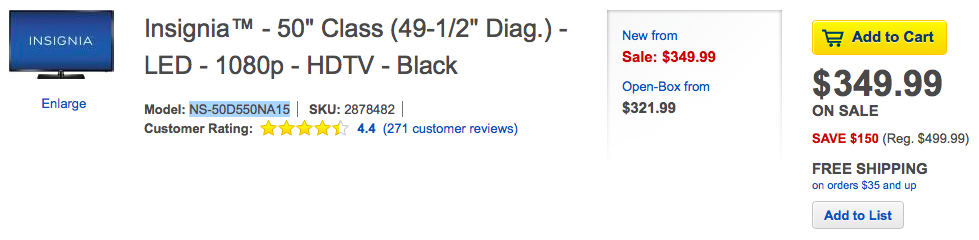The image appears to be a screenshot from an Amazon product page showcasing an Insignia 50-inch Class LED 1080p HD TV in black. On the left side of the image, there is a small picture of the TV, which can be enlarged by clicking the "Enlarge" option. The product is listed as new for $349.99, with an open-box option available for $321.99. There is a prominent "Add to Cart" button displaying the sale price of $349.99, highlighting a $150 discount from the regular price of $499.99. The page also mentions free shipping on orders of $35 and up. Additionally, there is a gray button labeled "Add to List" in blue print underneath the pricing details.